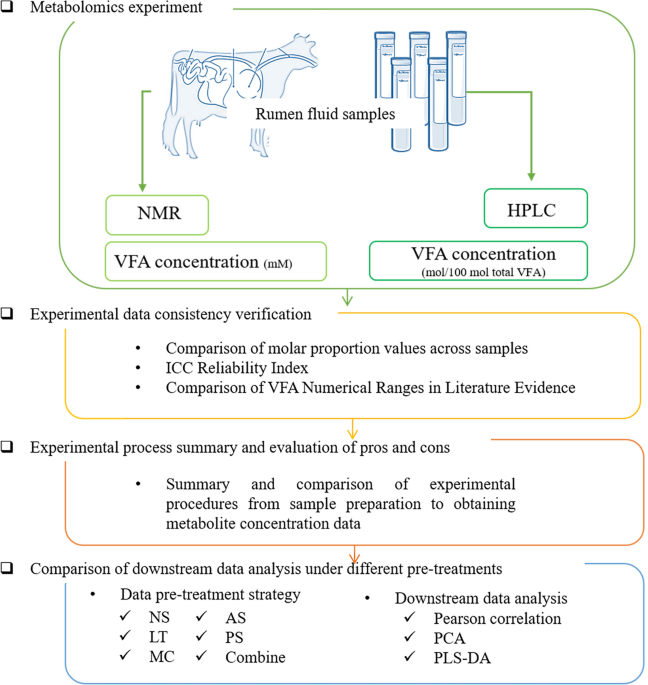The image is a detailed scientific flowchart explaining how to compare various values obtained from samples taken from a cow. The chart begins at the top with a checkbox labeled "Metabolomics Experiment," next to which is a pencil drawing of a cow showcasing its internal organs. Adjacent to the cow illustration, it mentions "Rumen and Fluid Samples" and depicts a set of five test tubes. An arrow extends downward from the test tubes to a box labeled "HPLC" and then "VFA concentration." 

Following this, a sequence of boxes stacked vertically leads the viewer through different stages of the workflow. The next box is labeled "Experimental Data Consistency Verification," followed by "Experimental Process Summary and Evaluation of Pros and Cons," and finally "Comparison of Downstream Data Analysis under Different Pretreatments." Each step in the process is connected by arrows, guiding the viewer through the stages of sample processing and data analysis, with the initial step indicating the necessity to check boxes one by one as each phase is completed.